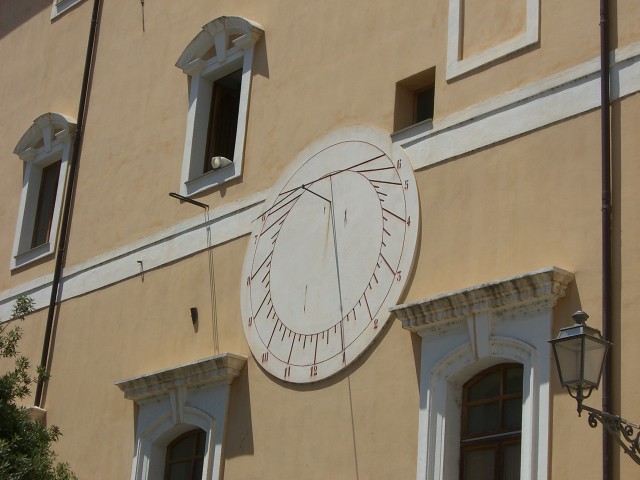The photograph captures the side view of an elegantly crafted sandstone building, bathed in warm, earthy tones. Diagonally across the structure, separating two visible floors, is a distinct white strip possibly made of wood or stone. Above this strip, two white-framed windows stand out, each capped with slightly ornate arches. The left window is shut, while the right window is open with what appears to be a white sock hanging out.

Below these, just the upper portions of two more arched windows are visible, mirroring the white frames and segmented into square panes, adding symmetry to the building's design. To the far right, a black pole runs vertically along the building’s facade, and in the bottom-right corner of the image, a traditional lantern-style street lamp adds a vintage charm to the scene.

Notably, a large, uniquely designed clock face stands out on the building. Its numbers appear upside down, suggesting it functions as a sundial. The clock displays "12" at the bottom, with numbers arranged anti-clockwise, from "1" to "5" along the left curve, and reappearing from "8" onwards to "11" on the right, leaving a gap at the top. This intriguing feature not only marks time but also adds a historical and artistic touch to the architectural beauty of the scene.